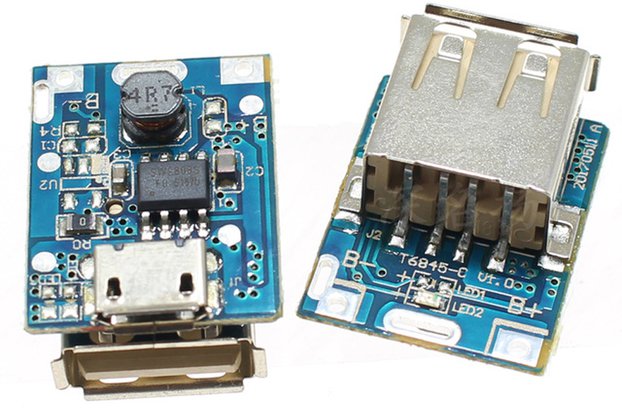The image portrays two intricate blue circuit boards positioned side by side against a stark white background. Each circuit board is adorned with various silver, black, and white connectors and components. On the left circuit board, a black segment with the inscription "4RV" is discernible, along with a metal port-like section along its front edge. The right circuit board features a prominent square silver module, approximately the size of a battery, with "AA" imprinted on it. Additional notable markings on this right board include "T6845C," "B minus," "B plus," and "LED1," "LED2." This module is secured with two clips and slightly angles to the right. The interconnected squares, rectangles, and lines on both boards highlight their complex design, indicative of essential components found within a computer's electronic system.